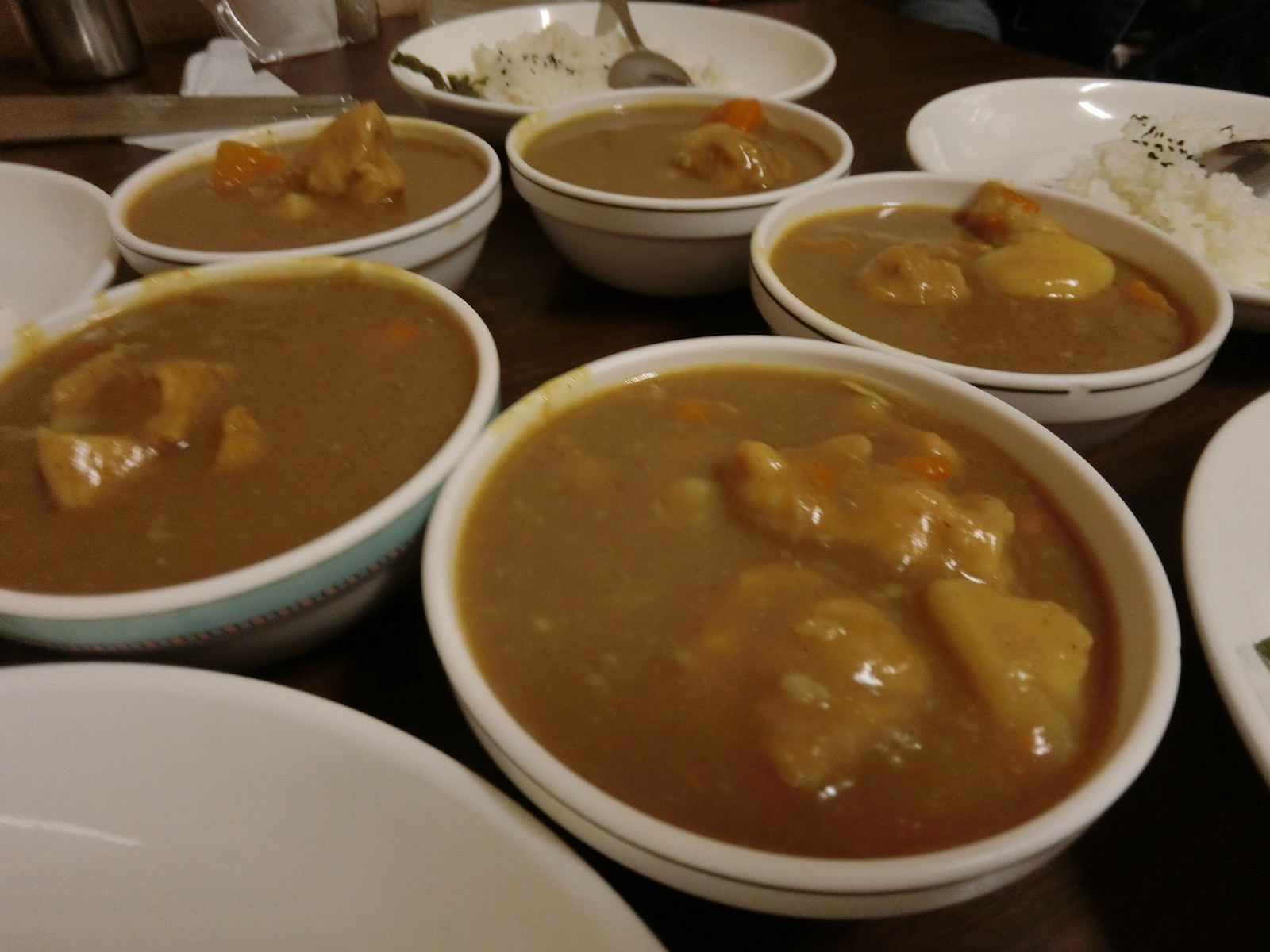The image showcases a detailed arrangement of approximately ten bowls and plates placed on a brown table. Central to the scene are five distinct bowls filled to the brim with a rich, gravy-like broth which appears to contain egg foo young. These bowls are predominantly designed with black rims, save for one unique bowl displaying a teal-colored rim. Surrounding these central bowls are five plain white bowls of similar size, each containing a serving of rice topped with black pepper or seeds, and accompanied by large spoons. Additionally, there are other partially visible white items around the edges of the image, although their exact nature isn't clear. The entire setup creates an inviting, well-organized presentation of the meal components, drawing attention both to the contrasting bowl designs and the harmonious pairing of the egg foo young and rice.